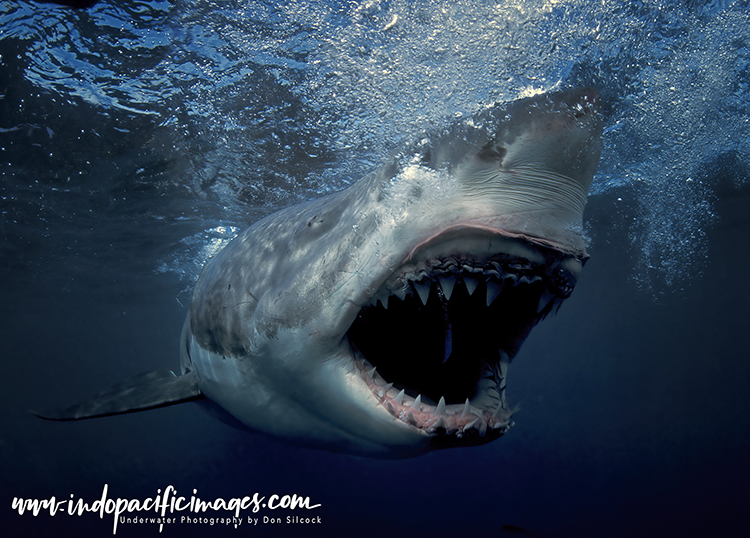In this underwater photograph, a massive great white shark dominates the frame, captured at a moment when its mouth is wide open, revealing its formidable, jagged teeth. The shark's upper body is a slate gray, while its underbelly and the area around its mouth are stark white. The image provides a clear view of the shark's menacing teeth, arranged in two rows on both the top and bottom jaws, with pink gums peeking through. The creature appears to be facing slightly to the right, and you can discern one of its fins, while the other remains unseen. The water is an intense deep blue, transitioning to a lighter shade near the surface where air bubbles rise and create a rippling effect. A single eye of the shark is visible, further adding to the ferocity of its appearance. In the bottom left corner, the text "www.indopacificimages.com. Underwater Photography by Don Silcock" is displayed in white font, attributing this striking image to the photographer.